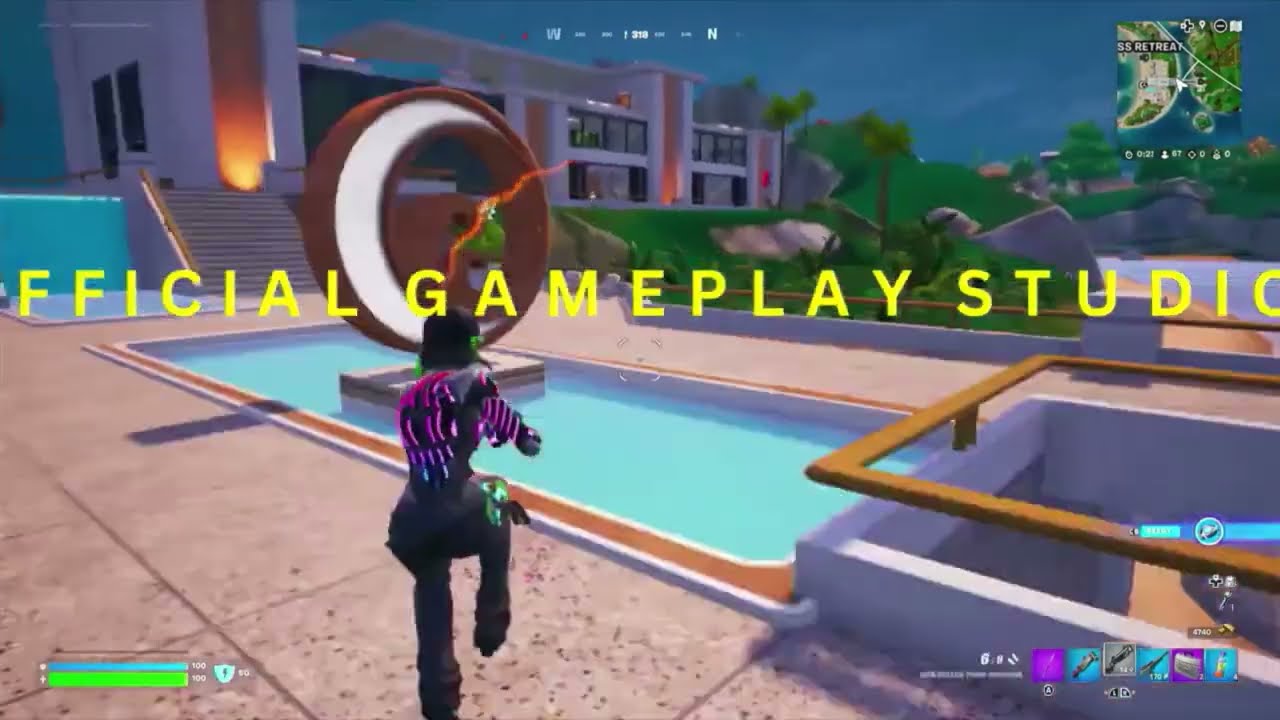The image is a detailed screenshot from Fortnite gameplay, showcasing a female character centered slightly to the left, wearing a distinctive jumpsuit with black pants, black boots, and a purple and blue striped shirt. The character also sports a black helmet and is positioned facing away from the viewer towards an in-ground pool. In the middle of the pool is a large spherical statue. Surrounding the pool is a grand mansion with numerous white columns and many windows, accessed by several stairs. This structure is set against a lush, green hillside.

The time appears to be transitioning from daytime to nighttime, and the scene is dimly lit. Overlaying the scene is the yellow text "Official Gameplay Studio," though the "O" in "Official" is missing, and the "O" in "Studio" is partially cut off.

In the top right corner of the screen is a minimap highlighting the current area, while the bottom corners display crucial game information: the bottom left shows the character’s health bar in green and armor in blue, with a small shield icon. The bottom right corner presents a variety of weapons to choose from. The overall ambiance is that of a tense, strategy-filled moment in the game.